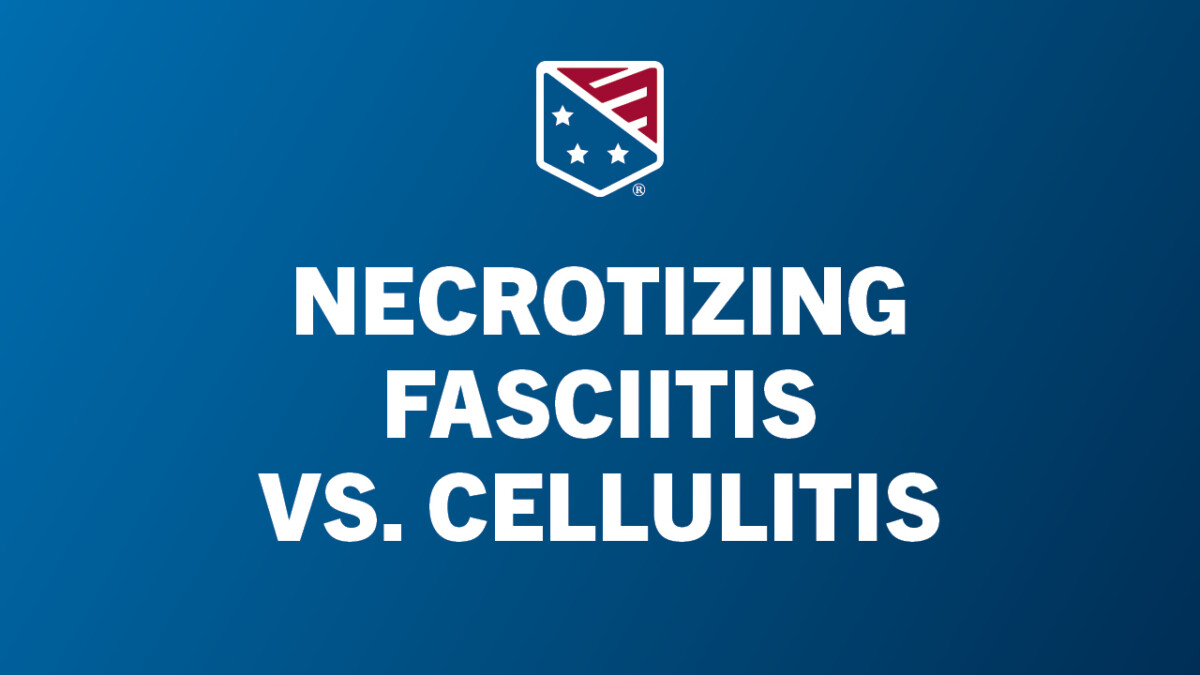This close-up image depicts a bold, informational slogan at its center with the text "Necrotizing Fasciitis versus Cellulitis" in prominent, white block letters against a medium to dark blue gradient background. At the top of the image, there is a logo resembling a modified chevron split into two sections: the left half features a blue background adorned with three white stars, while the right half displays a red background with three white stripes. The entire chevron is outlined in white. This logo appears to be associated with the slogan, which might suggest it is a company logo or emblem tied to the message being conveyed. The slogan is centrally positioned, ensuring that it is the primary focus of the image, with no other humans, objects, or text present to detract from it. The purpose of the image remains somewhat ambiguous, potentially part of a book, a poster, or some informational material, yet it clearly aims to highlight the differences between necrotizing fasciitis and cellulitis.